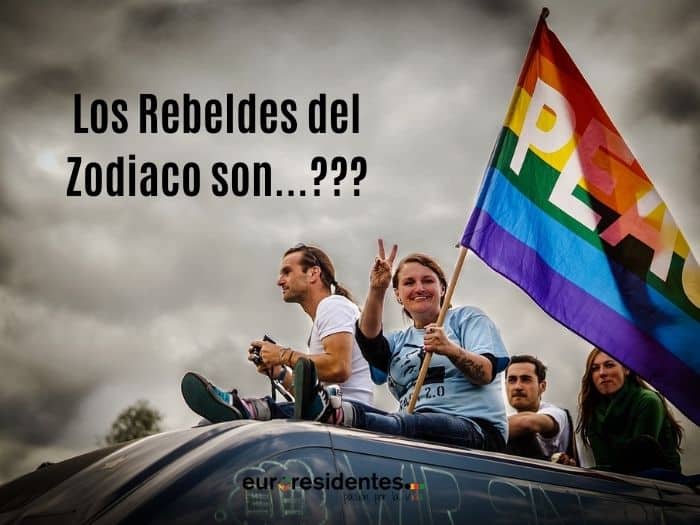In this evocative image set against a dark, cloudy, and stormy sky, four individuals sit on top of what appears to be a van, with a poignant message in black letters at the top left that reads, "Los Rebeldes del Zodiaco Son...???" The central figure is a woman with tattoos, dressed in a blue shirt with a graphic design. She is holding a rainbow-striped flag symbolizing peace, though only the letters "P," "E," partial "A," and the edge of "C" are visible. Her legs are extended out, black sneakers peeking out, as she faces the camera with a peace sign and a warm smile. Next to her sits a man with long hair tied in a ponytail, glasses, and a white t-shirt, holding a camera. Behind them is another man with short black hair and a white shirt, and a woman with long brown hair wearing a green long-sleeved shirt. The camera angle captures them from below, emphasizing their solidarity and the storm rolling in behind them, hinting at the fierce determination of a possible rally or peaceful protest.